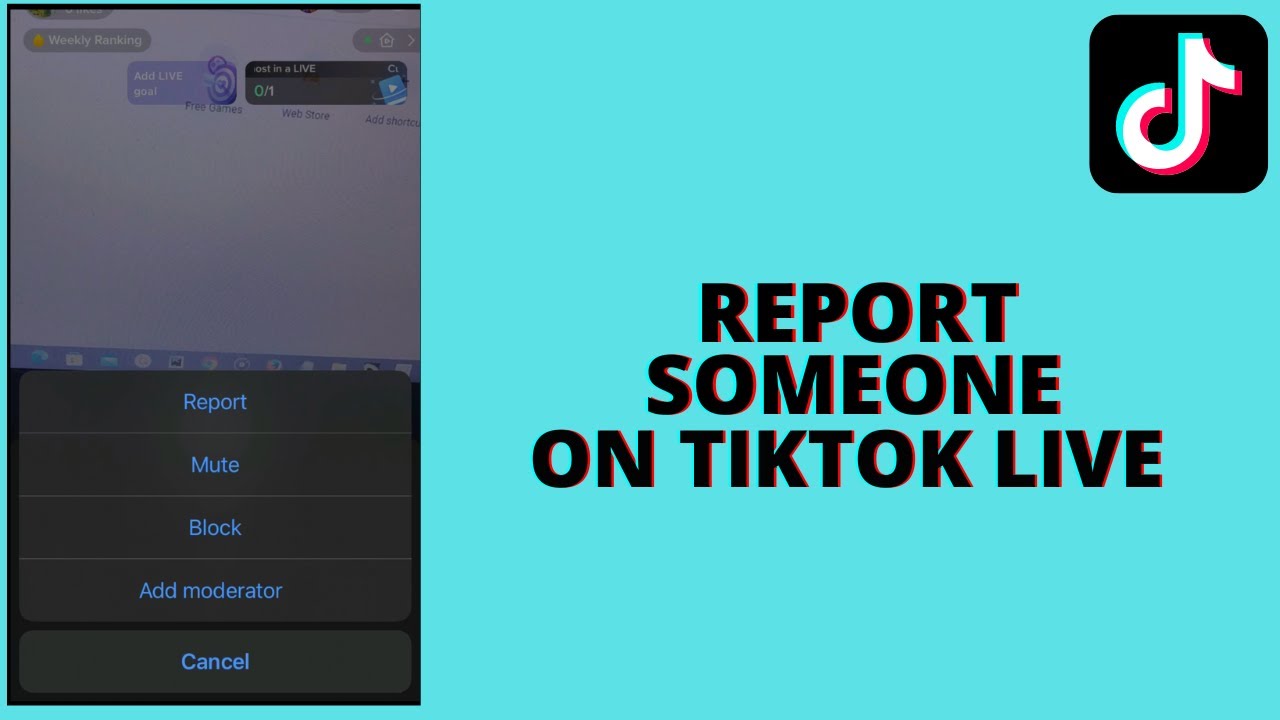The image's main focus is a bold message in the center that reads "Report Someone on TikTok Live" in striking black letters. The background is a vivid aqua blue, making the message stand out prominently. In the upper right corner, the recognizable TikTok logo is present, featuring a black circle with a musical note design that resembles a lowercase 'd' with a line extending from the top, colored in white with aqua blue and pink accents. The left side of the image is slightly darker, revealing two small chat boxes with indistinct text. Below these chat boxes, there are black rectangles with white text, each containing action options: "Report," "Mute," "Block," "Add Moderator," and "Cancel."